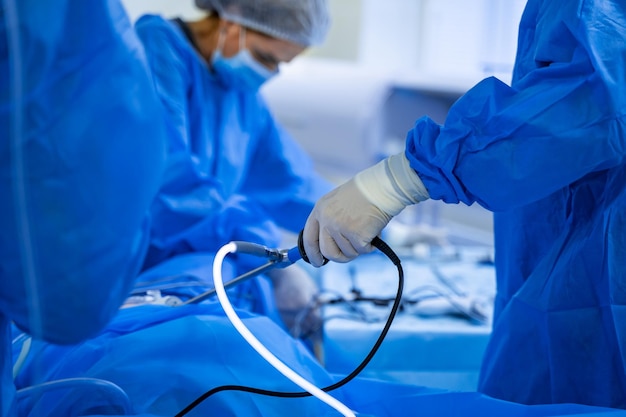The horizontally aligned rectangular image showcases a detailed scene from an operating room. Central throughout the image are several doctors engaged in a surgical procedure, all clad in blue scrubs and blue-and-white masks, with hairnets covering their heads. The scene is slightly blurry at the top but clearly shows a female doctor on the left, focused on her task with her hands busy. To the right, there is the left side of another medical professional's body, also in blue scrubs and white nitrile gloves, though their head and lower body are out of the frame. On the far left, only the back side of an arm and elbow of another person is visible. The patient lies in the center, almost entirely obscured by a blue drape. In the lower-left corner, a medical instrument with a silver tip held by the gloved hand is noticeable; it features both a black and illuminated white cord. The background, though blurred, hints at a multitude of surgical instruments laid out, emphasizing the clinical environment and the meticulous nature of the scene.